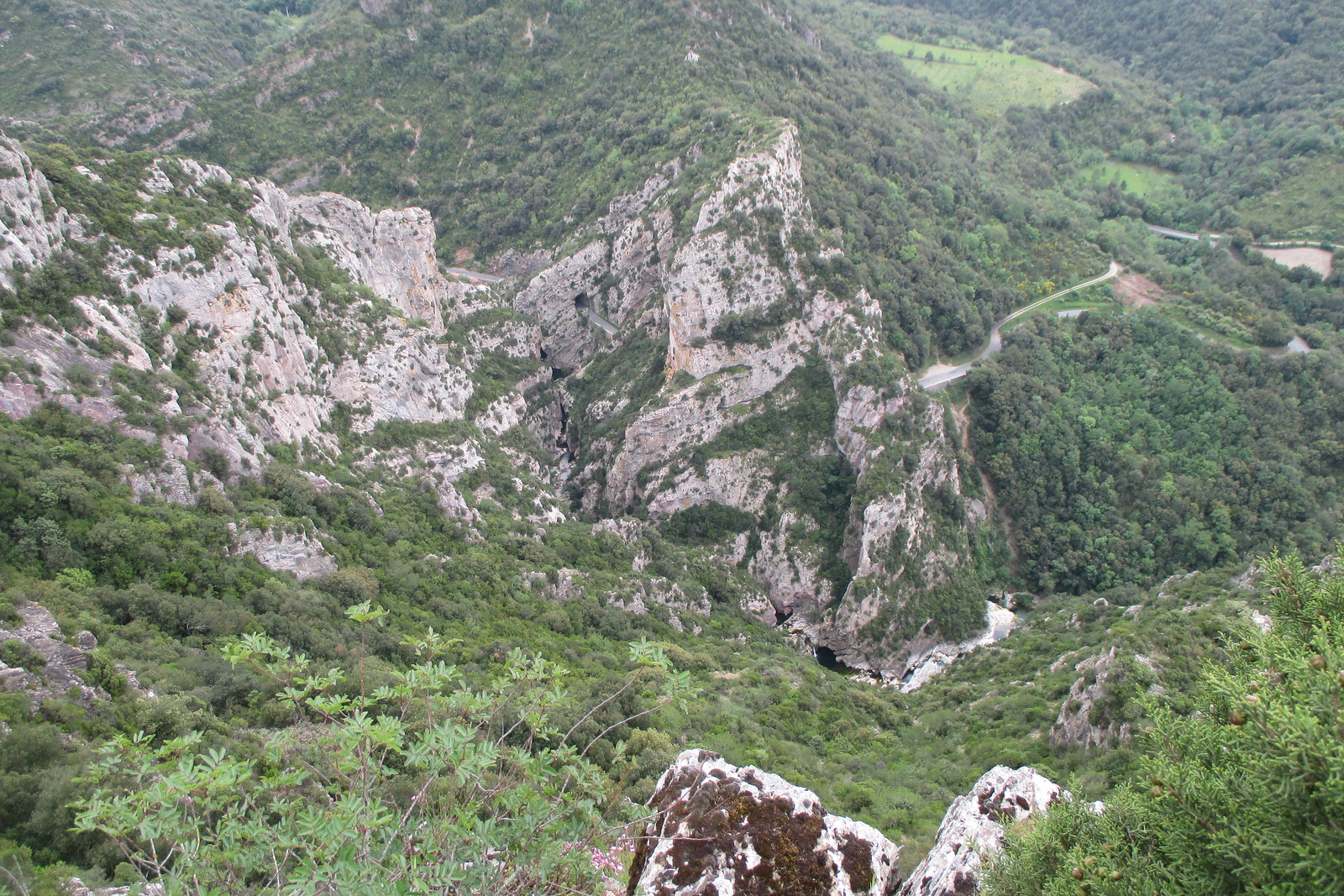This photo, taken from an elevated vantage point on a mountainous landscape, reveals a stunning vista of rugged terrain and verdant expanses. The foreground is characterized by rocky outcrops adorned with brown shrubs and grass, particularly noticeable in the bottom centers and corners of the image. From this high perspective, viewers can observe a large white mountain dominating the middle of the scene, its slopes transitioning from stark rocky surfaces to grassy inclines scattered with green shrubbery. 

In the center right of the photo, a winding road can be seen carving through the rocky landscape, leading downward and gradually disappearing off-screen. This road appears to connect to a grassy field devoid of trees further down, and possibly to a small body of water or river situated within the valley below. To the top left, the scenery extends into more mountainous terrain, peppered with trees and plants. The image richly captures the interplay between the rocky, rugged highlands and the lush, green valleys, presenting a breathtaking and detailed view of this natural landscape.